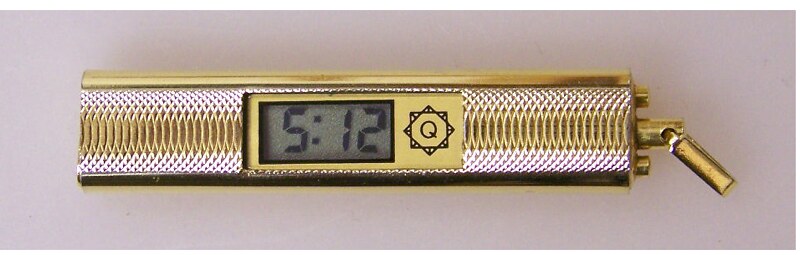This photograph captures an intricate digital clock encased within a longer, rectangular, golden keychain. The keychain features detailed texturing along its sides, with alternating silver and gold striped patterns accentuating the center. Adjacent to the digital clock face, a square star-shaped logo is prominently displayed, with a boldly drawn black "Q" at its center. The digital clock, set against a dark gray background, clearly reads "5:12" in black numerals. The entire keychain rests against a pink backdrop, which could be a piece of fabric, a table, or a desk, adding an appealing contrast to the golden hues of the keychain.